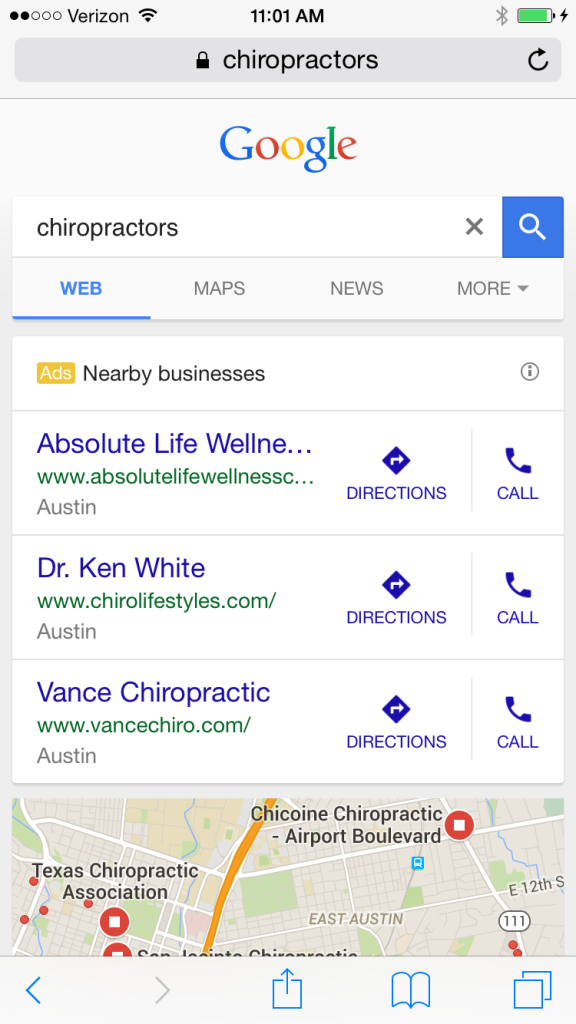A detailed screenshot of a Google search results page for the query "chiropractors." At the top of the image, the browser's address bar is visible, displaying the search URL. The address bar has a gray background. Below it, the Google logo is prominently displayed at the top of the page, followed by a white search bar that contains the query "chiropractors." To the right of the search bar, there is a blue search button.

Immediately beneath the search bar, there are four navigation links: "Web," "Maps," "News," and "More." Below these links, a yellow label indicates the presence of advertisements, with a tag reading "Ads, Nearby businesses." 

Under this label, there are three search results, each consisting of a blue title link, a green URL, and a gray location descriptor indicating "Austin." To the right of each result, blue buttons for "Directions" and "Call" are available.

The bottom section of the screenshot displays a map, providing a visual representation of the search results' locations.